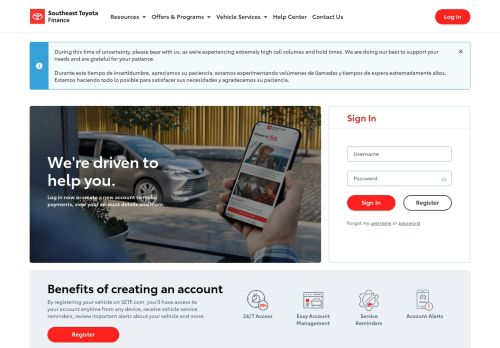This image is a slightly blurry screenshot taken from a laptop. It captures a webpage from Southeast Toyota Finance, organized into four main rows.

The top row features a white background with "Southeast Toyota Finance" positioned in the upper left-hand corner. To the right are navigation tabs labeled "Resources," "Offers and Programs," "Vehicle Services," "Help Center," and "Contact Us." In the upper right-hand corner, there is a prominent "Login" button.

The next section of the page has a light blue background and contains an important message regarding high call volumes and hold times due to current uncertainties. The message assures customers that the company is doing its best to support their needs and thanks them for their patience. This section likely continues in Spanish, with an option that allows users to close it.

Below this is a large outdoor image showing a car with a person standing in front, holding a cell phone, presumably accessing the app. To the right of this image is a sign-in box, which includes fields for logging in and both a red and a white login button.

The bottom row has a gray background and details the benefits of creating an account, illustrated with small icons. This row also features a red "Register" button located in the bottom left-hand corner.